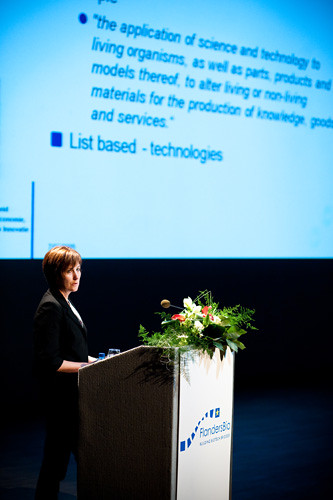In this image, a solemn-looking woman with short red hair is delivering a presentation at what appears to be a business or technology conference. She stands slightly to the left side at a podium adorned with a large bouquet of flowers. She is dressed in a black business suit with a white shirt. Behind her, a giant projection screen takes up the entire top half of the photograph, displaying detailed information about the application of science and technology to living organisms, parts, products, and models, with the aim of altering living or non-living materials for the production of knowledge, goods, and services. There is a white sign with light blue lettering on the front of the podium that includes a corporate logo, though the text is too small to read. The overall setup indicates that the woman is engaged in a formal presentation to a crowd.